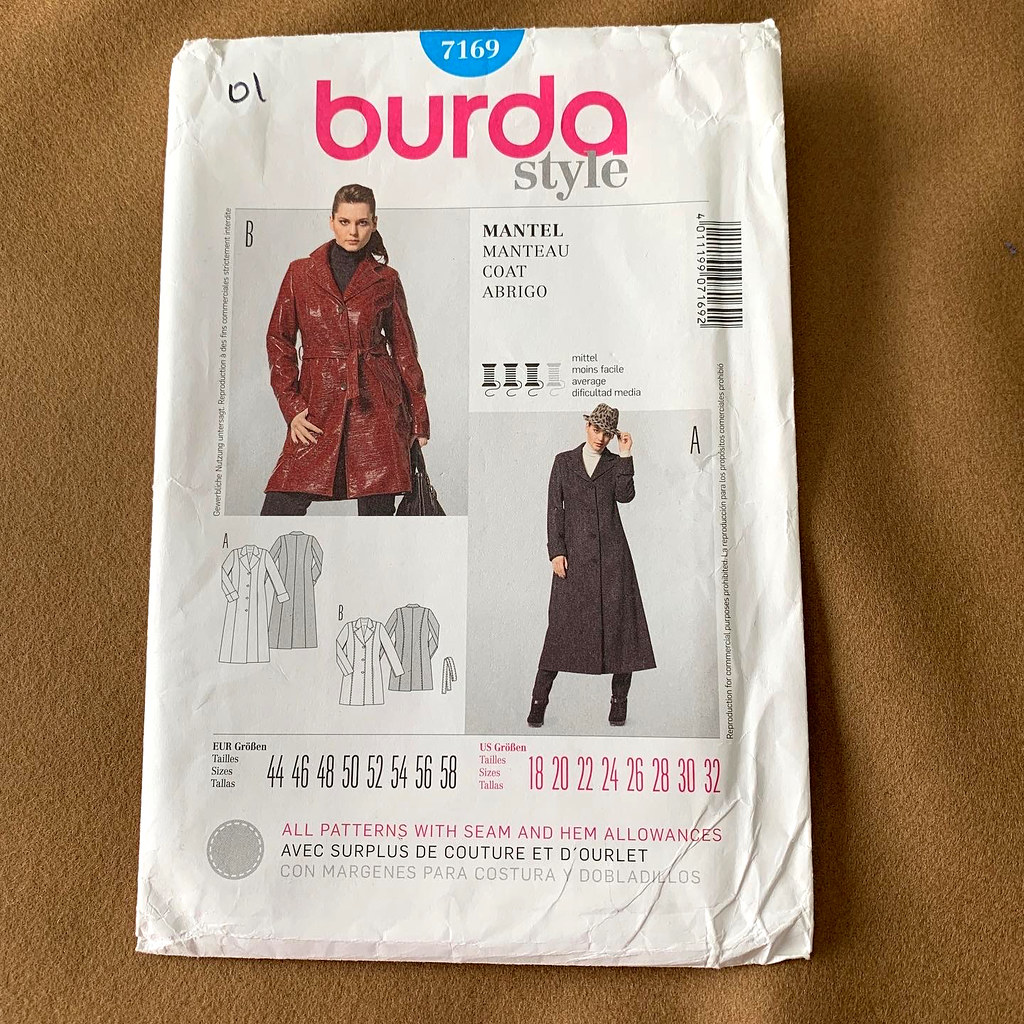The image features a rectangular white envelope, approximately eight by three inches, resting on a surface covered with brown fabric. The envelope showcases a clothing pattern package. At the top, a blue semicircle contains the number "7169" in white font. Below this, in bold pink letters, it reads "BURDA," with the word "style" in gray underneath.

In the center of the envelope are two photographs of models wearing trench coats, labeled with the caption "Mantel-Monteau-Coat-Abrigo." The model on the top left is wearing a shorter, red coat, while the model on the bottom right is in a longer, gray jacket. Additionally, to the left of the images, there are black and white illustrations of the coat patterns. The background fabric is brown, framing the entire scene. The packaging clearly emphasizes the patterns available for creating these coats, including seam and hem allowances. 

Overall, this packaging provides a detailed overview of two different trench coat styles, aiming at DIY sewing enthusiasts.